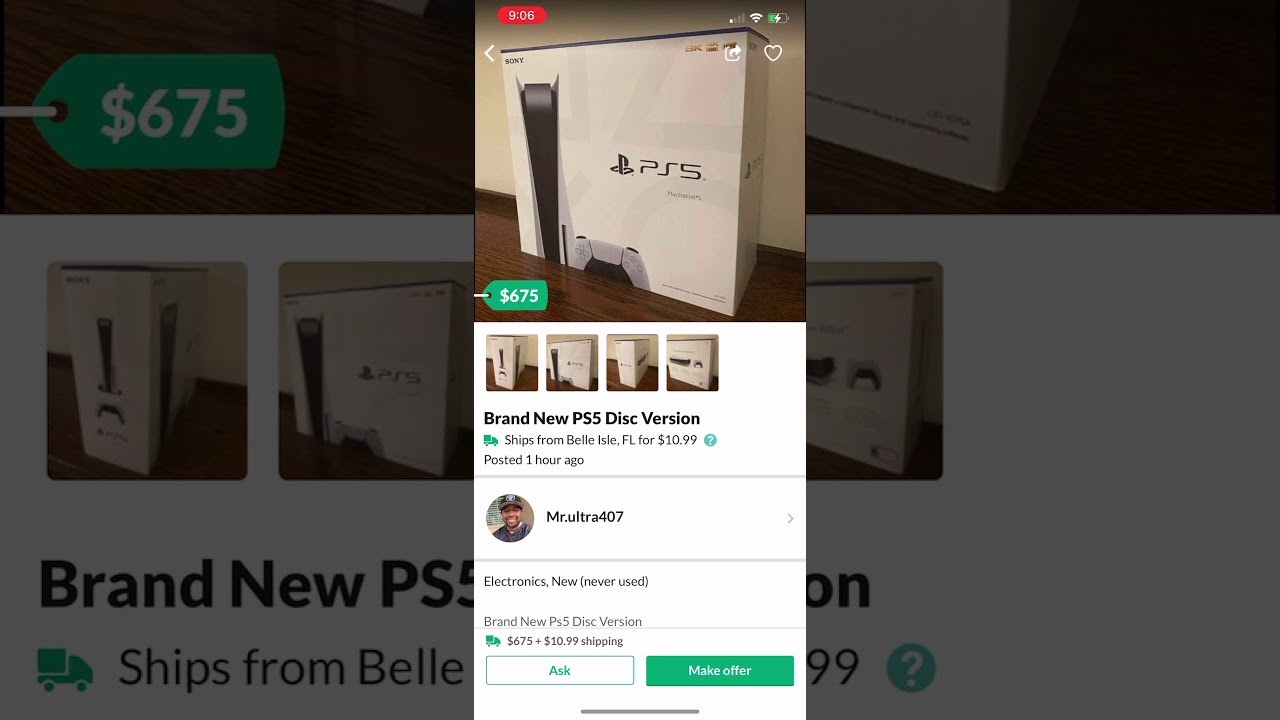In this landscape-oriented image, the background displays a webpage where an individual is browsing to purchase a PS5. The webpage has a darkened theme on the left side, showing a green label with the price "$675" in white script. This label extends off the left edge of the image and is placed against a black horizontal banner. Above this banner, the top portion reveals a white PS5 box.

Below the banner, a white section displays three to four photographs of the PS5 in its box, captioned "brand new PS5." However, part of this section is obscured by a pop-up on the screen, making the full text difficult to read. A green truck icon accompanies text indicating the item ships from Bell Isle, FL, for $10.99. There is also a partially visible green icon with a white question mark.

The pop-up itself, in portrait orientation, provides a clearer view of the listing details. This smaller version of the webpage prominently features a white PS5 box on a brown table, four additional square photos of the PS5 and its packaging, and the text "brand new PS5 disc version, ships from Bell Isle Florida for $10.99, posted one hour ago" by user MrUltra407. This user’s avatar, placed to the left of their name, depicts a smiling black man in a black baseball cap.

Underneath the main heading, the listing specifies "electronics, new, never used" and reiterates the condition and pricing: "brand new PS5 disc version, $675 plus $10.99 shipping." Two interactive buttons are shown: an "Ask" button (green text on a white background) and a "Make Offer" button (white text on a green background).

Overall, the main image is amplified by the pop-up, which details the same content but in a condensed, more readable format, ensuring the essential information about the PS5 listing is highlighted despite the background clutter.